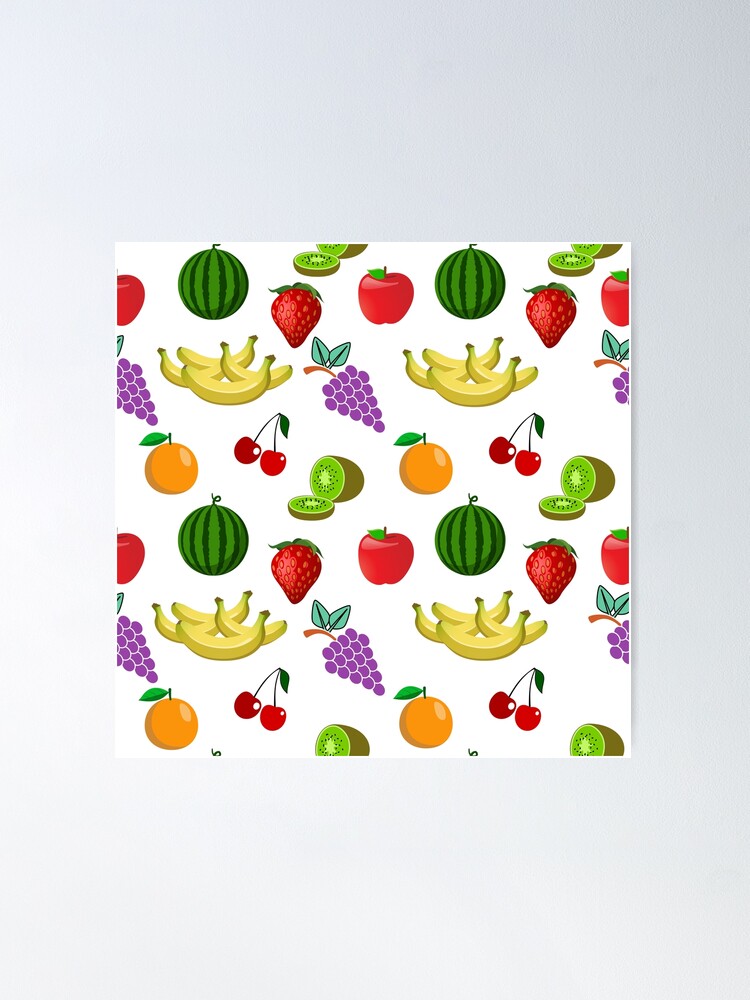The image features a colorful and detailed fruit collage set against a sleek, metallic background that gradients from dark gray on the right to light white on the left. The central pattern displays an orderly assembly of various fruits including a green watermelon, red strawberries, purple grapes, red apples, yellow bananas, oranges, shiny red cherries, and green kiwi slices. The pattern starts with an apple, followed by a watermelon to its right, then a strawberry below the watermelon. Above the strawberry and slightly to the right is a kiwi, with four crossing bananas situated directly below the watermelon. A bunch of grapes is positioned to the left of the bananas, an orange sits at the bottom of the grapes, and two cherries are found to the right of the orange. This arrangement repeats seamlessly in a tiled manner, covering the central section of the image without occupying more than half of the total image space. The fruits are meticulously placed to ensure the pattern's noticeable repetition, contributing to a vibrant yet orderly visual appeal.